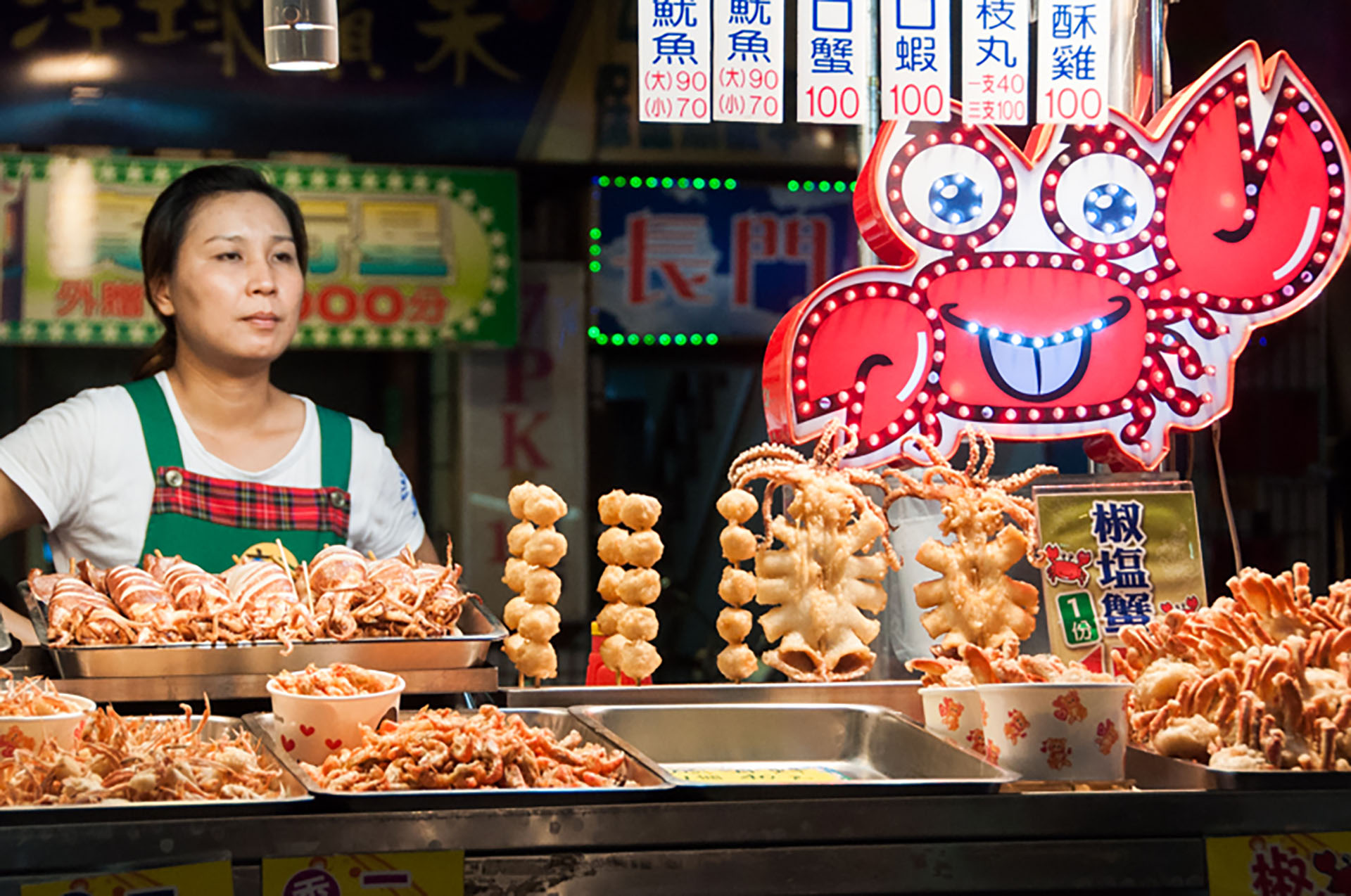The image captures a vibrant food vendor stall likely located in Japan or China, as suggested by the foreign text, predominantly in Chinese characters, seen on various signs and hoardings in the background. This stall is part of what appears to be a bustling food event or market, with lights and advertisements enhancing the lively atmosphere.

The focal point of the image is a food counter adorned with a lighted animated cartoon crab logo, clearly indicating the specialty of the vendor. Above the logo are price tags written in Chinese, with numbers like 90, 70, and 100 prominently displayed. At the counter, a woman of Asian descent, with black hair, stands attentively. She is dressed in a white t-shirt and a green apron, overseeing an array of delectable food items arranged in trays and buckets, mostly fried and grilled.

The vivid colors of reds, blues, whites, greens, yellows, beiges, and blacks blend harmoniously, creating an inviting and colorful scene. To the right of the counter, you can see the animated crab logo alongside the prices, while the different types of food are displayed below it. In contrast, the left side features the woman overseeing the food, with a view of more advertisements and a dimly lit hallway further enhancing the market's atmospheric depth.